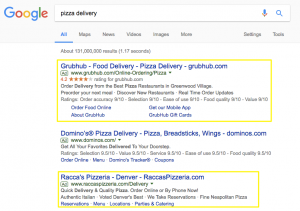The screenshot captures a Google search page with visible search results. The image is somewhat blurry and not of high resolution. 

At the top left corner, the Google logo is displayed against a very light gray background strip. The search bar is prominently placed at the top of the page, showing the search query "pizza delivery" typed in black text. To the right of the search bar, a microphone icon and a search icon are visible. 

Below the search bar, there are several tab options including "All," "Maps," "News," "Videos," "Images," and "More," with "All" highlighted in blue text and underlined, indicating it is the selected tab. To the far right, "Settings" and "Tools" options are also displayed.

The page indicates approximately 131 million results generated in 1.17 seconds. The search results display multiple advertisements related to pizza delivery services. 

The first ad is for Grubhub, highlighting food and pizza delivery services available at Grubhub.com, specifically suggesting it serves the Greenwood Village area. Additional links within the ad include "Order Food Online," "About Grubhub," "Get Our Mobile App," and "Grubhub Gift Cards." This ad is enclosed in a rectangle with yellow borders.

Below the Grubhub ad, a Domino's ad appears, promoting Domino's pizza delivery, breadsticks, and wings available at dominos.com.

The final ad in the screenshot is for "Rackers Pizzeria" in Denver, accessible at rackerspizzeria.com.